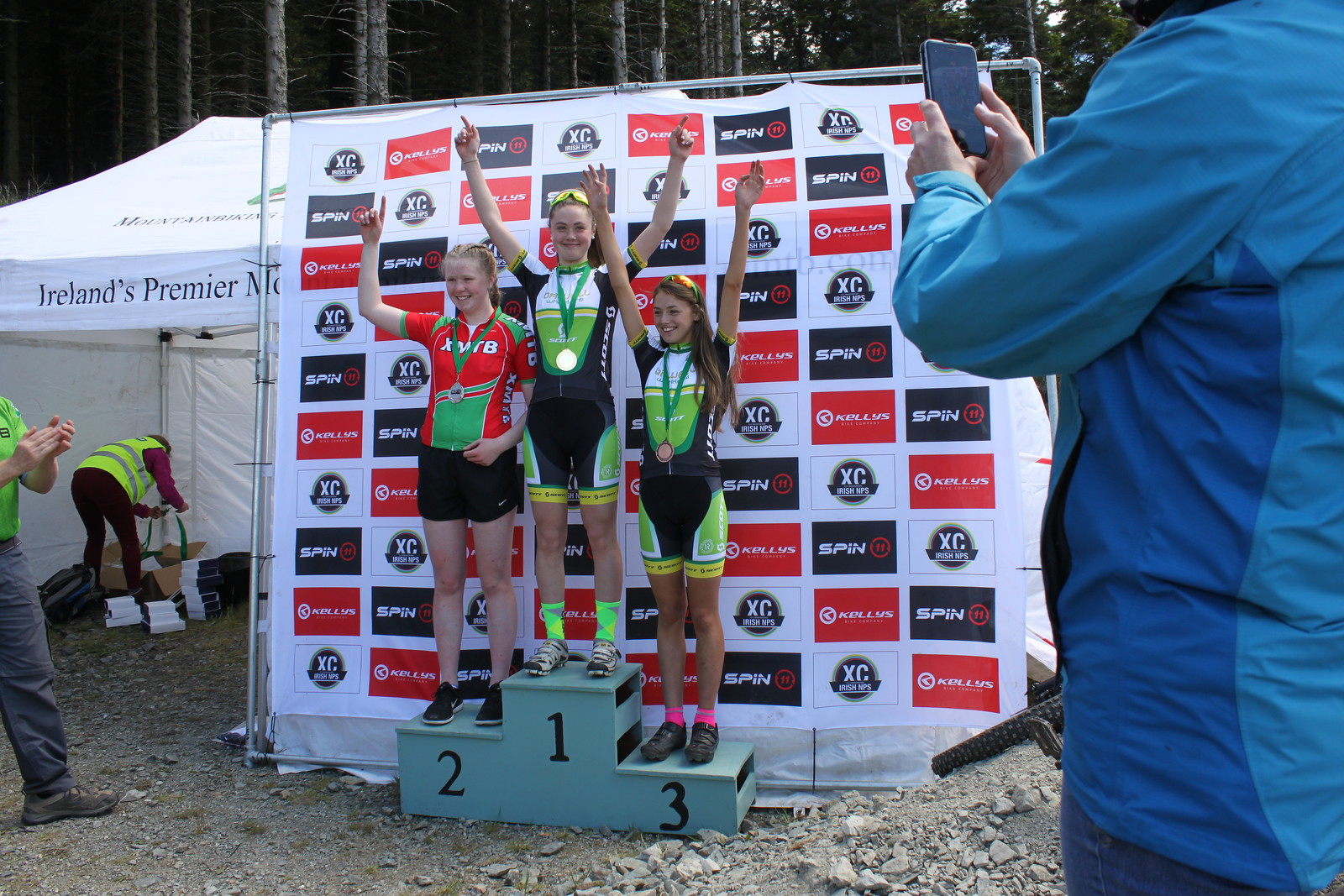The image captures the triumphant moment at the end of a race, likely a running event or a biking race, featuring three young women standing on a makeshift gray-blue podium against a checkered backdrop with advertising logos like "Kelly's" and "XC Irish." The podium, labeled distinctly with black numbers "1," "2," and "3," showcases the winners. Center stage on the tallest section, the first-place winner sports a black suit with green and yellow trim, black knee-length shorts, and bright green socks. She proudly raises both hands, signaling she's number one as her bright gold medal glistens against her chest. On the left, the second-place holder, dressed in a red jersey and black shorts, smiles while mimicking the number one with her right hand and resting her left across her belly. To the right, standing on the lowest section for third place, another girl donning an identical outfit to the first-place winner, with long hair cascading over her shoulders, lifts both hands energetically. The scene is set outdoors on a gravelly terrain with a white tent labeled "Ireland's premier" partially visible to the left, complemented by a person in a yellow safety vest and another, in a blue jacket on the right, capturing the joyous moment on their cell phone. Amidst this celebration, spectators and other individuals, including a clapping man, add to the vibrant atmosphere of achievement.